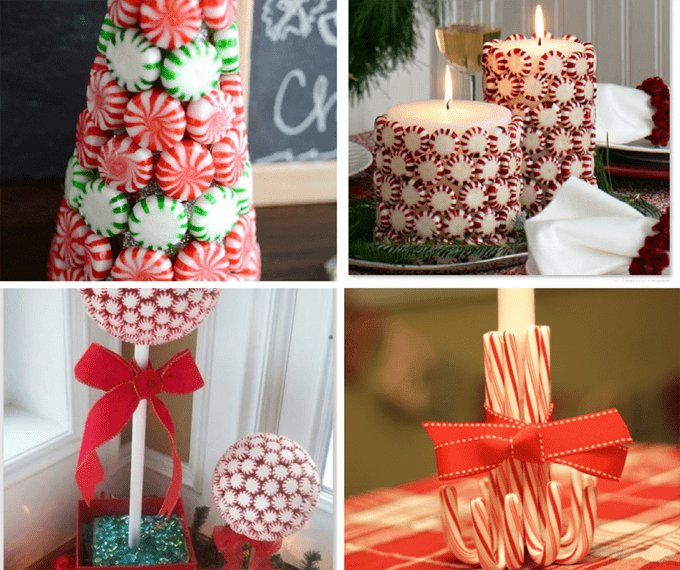This image is a collage of four festive holiday crafts, each creatively using peppermint candies. In the top left quadrant, there's a cone-shaped Christmas tree adorned with alternating stripes of red and green peppermint candies, giving it a joyful seasonal appearance. The top right quadrant showcases two large, white candles surrounded by red peppermint candies, forming a festive and aromatic outer casing. Moving to the bottom left, the image features a decorative topiary made from red and white peppermint candies, complete with a red bow, resembling a lollipop. Finally, the bottom right quadrant displays a unique arrangement of upside-down candy canes, bound together with a red ribbon and encircling a central candle, adding a charming touch to the holiday decor.